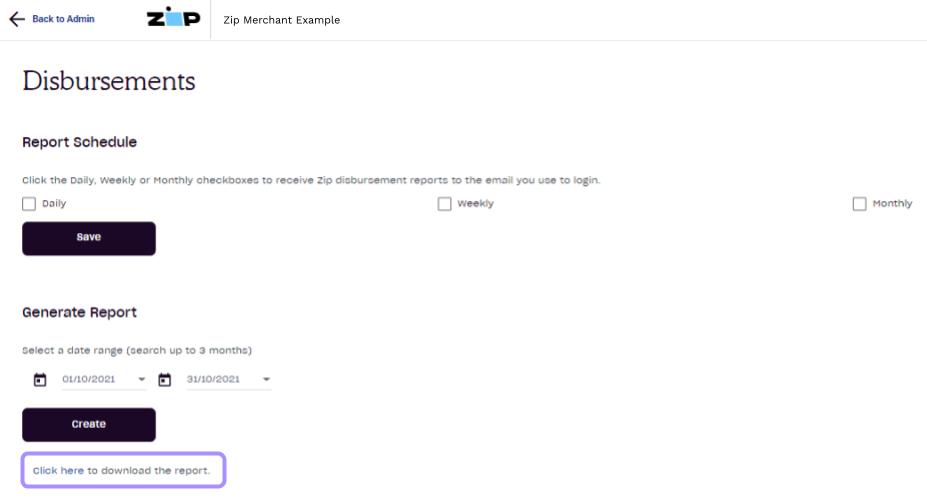The image features a clean white background with black text positioned in the upper left-hand corner. A leftward-pointing arrow accompanied by the text "Back to Admin" is prominently displayed. To its right, the word "ZIP" appears, followed by "ZIP Merchant Example."

Below this header, the title "Disbursements" is presented, under which "Report Schedule" is written. The instructions state: "Click the daily, weekly, or monthly check boxes to receive ZIP disbursement reports to the email you use to log in." Three selectable options labeled "Daily," "Weekly," and "Monthly" are displayed beneath these instructions, alongside a "Save" button.

Further down, under the "Generate Report" section, the text directs users to "select a date range (search up to three months)." An example date range "1-10-2021 to 1-10-2021" has been entered. A black "Create" button is positioned immediately below the date range input fields.

In the bottom left corner, there is a button outlined in purple that reads "Click Here to Download the Report." The rest of the right side of the image remains blank, with no additional images or text.